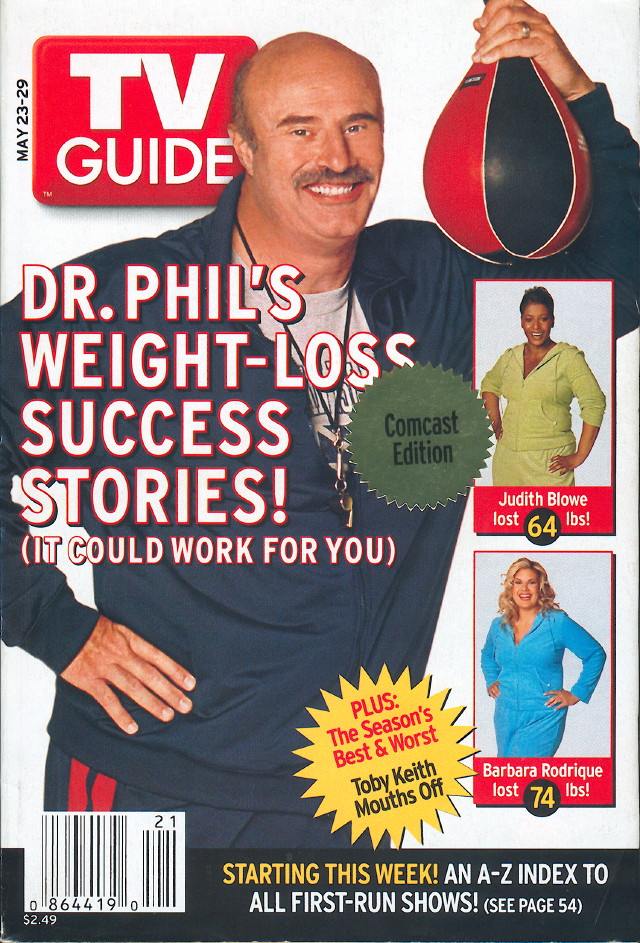This detailed magazine cover description for TV Guide captures all the notable elements and styling:

"TV Guide Magazine Cover – May 23rd to 29th Edition

The magazine cover is rectangular with a predominantly white background. A thin black rectangle at the bottom contains a barcode and the price, marked in white text, $2.49. Additionally, the bottom of the cover mentions 'A to Z, first run shows'. 

In the upper left corner, the TV Guide logo is prominently displayed in white text within a red rectangle. Just below the logo, the date of the magazine issue, 'May 23rd to 29th,' is printed.

Dr. Phil graces the cover, depicted in a gym trainer's outfit. He is holding a speed bag in one hand and wearing a whistle around his neck, suggesting a coach or fitness trainer persona. The main headline reads, 'Dr. Phil's Weight Loss Success Stories – It Could Work for You.'

On the front, a gold sticker denotes that this is the 'Comcast Edition.' A smaller, yellow sticker informs readers of additional content: 'Plus the Season's Best and Worst.'

Two pictures of women are located on the right side of the cover, next to another headline, 'Toby Keith Sounds Off.'

The cover art is meticulously laid out to capture attention and convey a range of engaging stories and features inside the magazine."